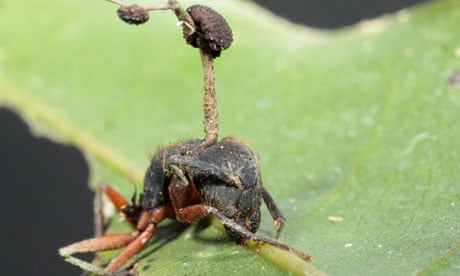In the image, an insect that resembles a cricket is prominently featured. This insect has a black, somewhat dirty-looking, hard-shelled body with reddish legs. Notably, the insect possesses a very long neck extending to its head, which is adorned with what might be antennae or sensory appendages sticking up like stems. These stems appear to have black clumps or egg sacs attached to them. The insect is perched on a vibrant green leaf, which shows signs of being chewed, possibly by this insect or others, as it has pieces missing. The leaf stands out clearly against a blurred, out-of-focus background. Additionally, there is a black blob in one corner of the image, contributing to the dark and detailed depiction of the insect and its surroundings. The description of the insect's legs includes two in the front, two on the side, and two at the back, bending much like grasshopper legs. The overall image captures the intricate details of this black-bodied insect and its natural habitat.